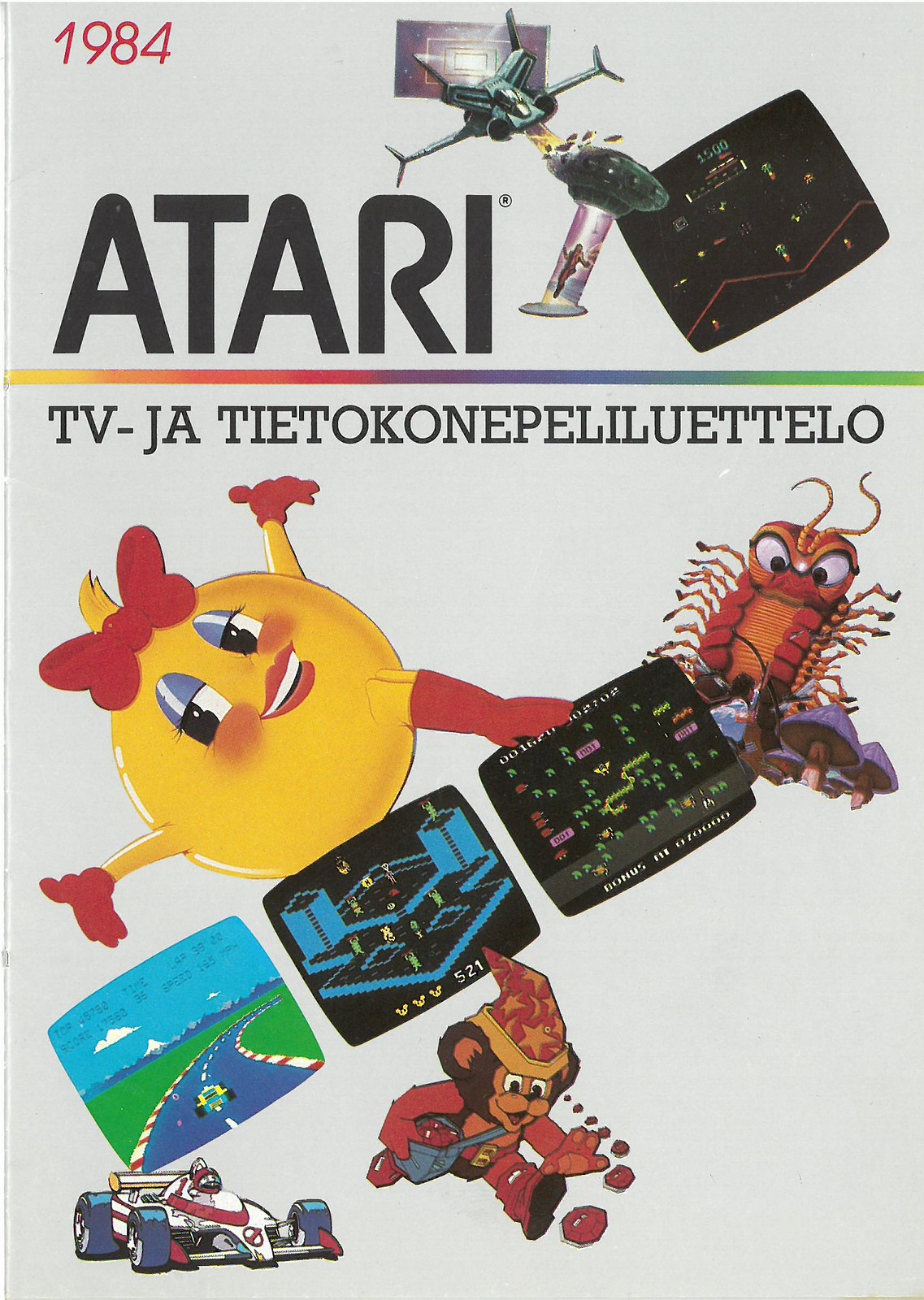The image features text and artwork on a light gray background. In the top left corner, "1984" is written in bold red letters. Directly below, "Atari" is spelled out in black. Below that, there is a line of text reading "TV-JA TITTIETOKONEPELI-LUETTEL-O." Above the "Atari" text is a green spaceship, and below it is another circular green spaceship. Further down the image, there is a shining figure of a person positioned to the right side.